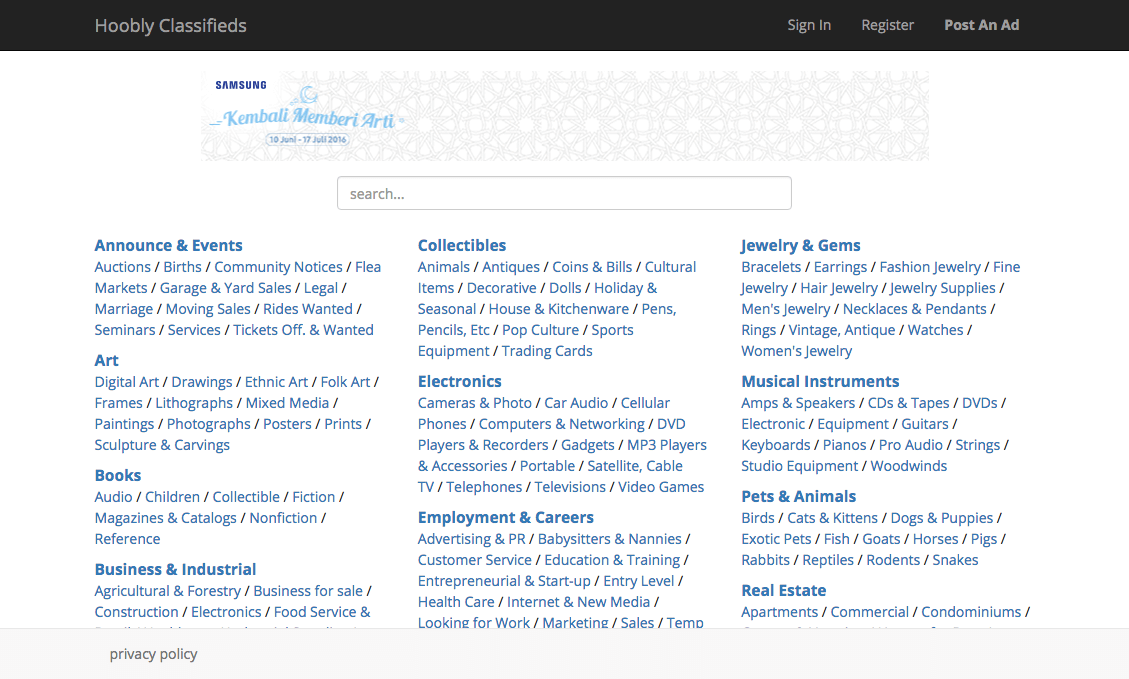The image depicts a black-themed website interface with an emphasis on a variety of classified sections. On the left side of the image, in grey text, the title "Hobby Classifieds" is prominently displayed. Adjacent to this, on the right side, there are clickable sections labeled "Sign In," "Register," and "Post an Ad," also in grey text.

In the central part of the layout, a white rectangular area showcases the brand name "Samsung" in dark grey and dark blue text. Below this, there's a light blue crescent moon icon and the light blue text "K-E-M-B-A-L-L." The text "Manverny" follows, with "R-T" and a complex string "M-E-M-B-E-R-I-A-R-T-I" also present within this area.

Further down, a rounded rectangle contains the text "10 June (7 July 2016)" along with a plethora of text beneath a search bar marked by three dark grey ellipses.

The website's content is divided into various headers and categories, each highlighted in bold blue text. The main sections include:

1. **Announcements and Events:**
   - Actions, Verse, Community Notices, Flea Markets, Garden and Yard Sales, Legal, Marriage, Moving Sales, Rides Wanted, Seminars, Services, Tickets Off, and Wanted.

2. **Art:**
   - Digital Art, Drawings, Electronic Art, Ethnic Art, Folk Art, Frames, Lithographs, Mixed Media, Paintings, Photographs, Posters, Prints, Sculptures, and Carvings.

3. **Books:**
   - Audio, Children, Collectibles, Fiction, Magazines and Catalogs, Nonfiction, and Reference.

4. **Business and Industrial:**
   - Agricultural and Forestry, Business and Sale, Construction, Electronics, Food and Service.

5. **Collectibles:**
   - Animals, Antiques, Coins and Bills, Cultural Items, Decorative Dolls, Holiday and Seasonal, Household and Kitchenware, Pens, Pencils, ETC, Pop Culture, Sports Equipment, Trading Cards.

6. **Electronics:**
   - Cameras and Photo, Car Audio, Cellular Phones, Computers and Networking, DVD Player and Recorders, Gadgets, MP3 Players and Accessories, Portable, Satellite, Cable TV, Telephones, Televisions, Video Games.

7. **Employment and Careers:**
   - Advertising and NPR, Babysitters and Nannies, Customer Service, Education and Training, Entrepreneurial and Startup, Entry-Level, Healthcare, Internet Media, Looking for Work, Marketing, Sales, Temporary Positions.

8. **Jewelry and Gems:**
   - Bracelets, Earrings, Fashion Jewelry, Fine Jewelry, Hair Jewelry, Jewelry Supplies, Men's Jewelry, Necklaces and Pendants, Rings, Vintage and Antique, Watches, Women's Jewelry.

9. **Musical Instruments:**
   - Amps and Speakers, CDs and Tapes, DVDs, Electronic, Equipment, Guitars, Keyboards, Pianos, Pro Audio, Strings, Studio Equipment, Woodwinds.

10. **Pets and Animals:**
    - Birds, Cats and Kittens, Dogs and Puppies, Exotic Pets, Fish, Goats, Horses, Pigs, Rabbits, Reptiles, Rodents, and Snakes.

11. **Real Estate:**
    - Apartments, Commercial, and Condominiums.

The detailed interface design creates a structured and navigable platform for users to explore classified ads across numerous categories.